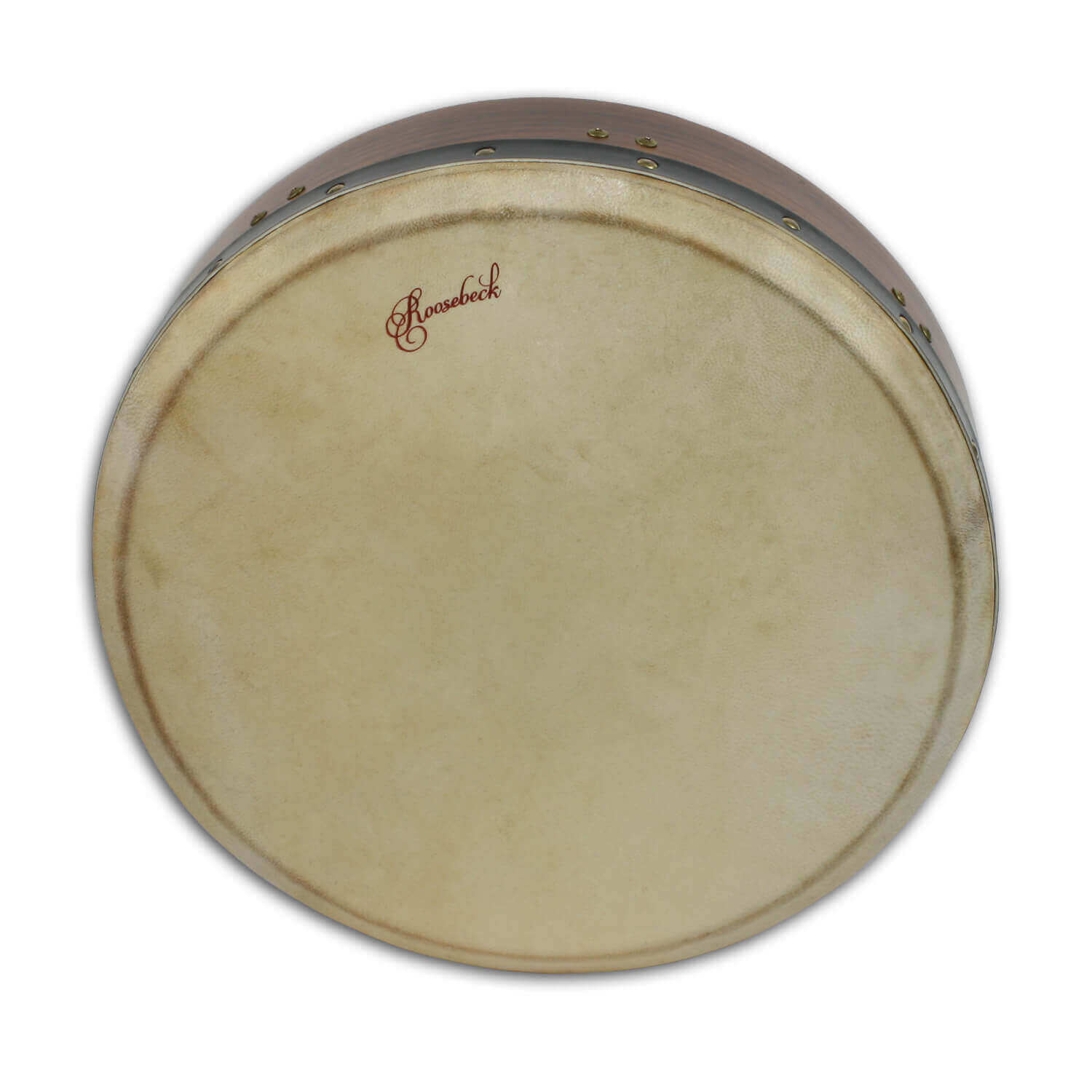The image features a close-up view of a well-worn drum, primarily showcasing its circular top. The drum head is a white, sheepskin-like membrane, but it shows signs of heavy use with brown and yellow discoloration. The drum's base is constructed from wood, and it's reinforced by metal rivets attaching a black ring that holds the drumhead in place. The wooden parts display a dull, brown finish that adds to the instrument's aged appearance. A red script logo, "Roosebeck," is prominently etched on the drumhead, adding an elegant touch with its old-fashioned font. There are no discernible background elements, making the drum the primary focus of the image.